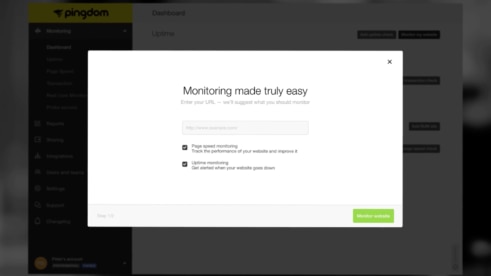This image captures a desktop-sized web page displaying a prominently centered, large white pop-up with a bold border. The pop-up features a headline in black lettering that reads, "Monitoring Made Truly Easy." Below the headline, there is additional text and a text input field, although these elements are too blurry to discern clearly.

The background of the web page is grayed out, but the title "Pingdom" is still visible, presented within a small yellow banner with bold black text. Adjacent to the Pingdom logo, which resembles either an upside-down triangle or a tornado, lies a navigation menu that cannot be clearly read from this image.  

To the right of the navigation menu, a grayed-out white web page is displayed featuring a title at the very top reading "Dashboard." The rest of the content on this page is indistinguishable. Additionally, there are small black boxes that likely serve as clickable options, though the text within these boxes remains unreadable.